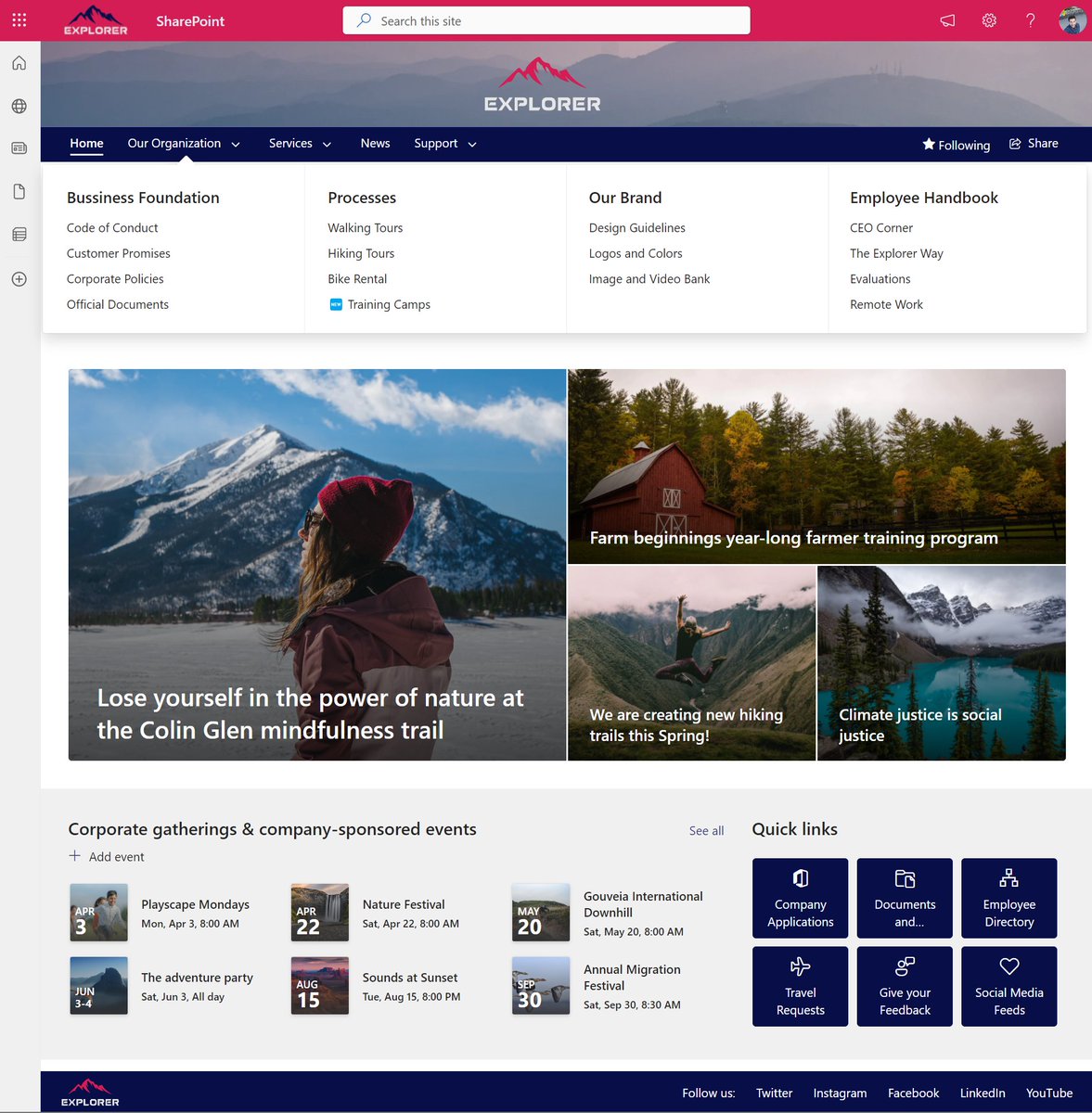Screenshot Description: 

The image is a detailed screenshot from a mountain exploration or vacation website, displayed on a widescreen or desktop device based on its formatting and layout. The website interface is dominated by a top navigation bar featuring a main address and search bar. The website's branding includes a stylish mountain logo positioned to the left.

Directly beneath the navigation bar, there's a striking magenta banner bearing the words "EXPLORER" in bold, white uppercase letters. Adjacent to the logo, the bar includes the text "SharePoint" along with an address bar situated centrally.

Further down, the website's branding is reiterated with another "EXPLORER" logo in which the mountain icon is rendered in pink. This logo is set against a backdrop of slightly hazy mountain imagery, evoking a sense of serene adventure.

Below this, a navy blue menu bar stretches across the screen, with white text indicating various sections: HOME, OUR ORGANIZATION, SERVICES, NEWS, and SUPPORT. The "OUR ORGANIZATION" section seems to be active, as evidenced by the visible drop-down menu. On the right side of this menu bar, there are several icons and labels, including a star icon followed by the word "FOLLOWING," and another unidentified arc icon accompanied by the word "SHARE."